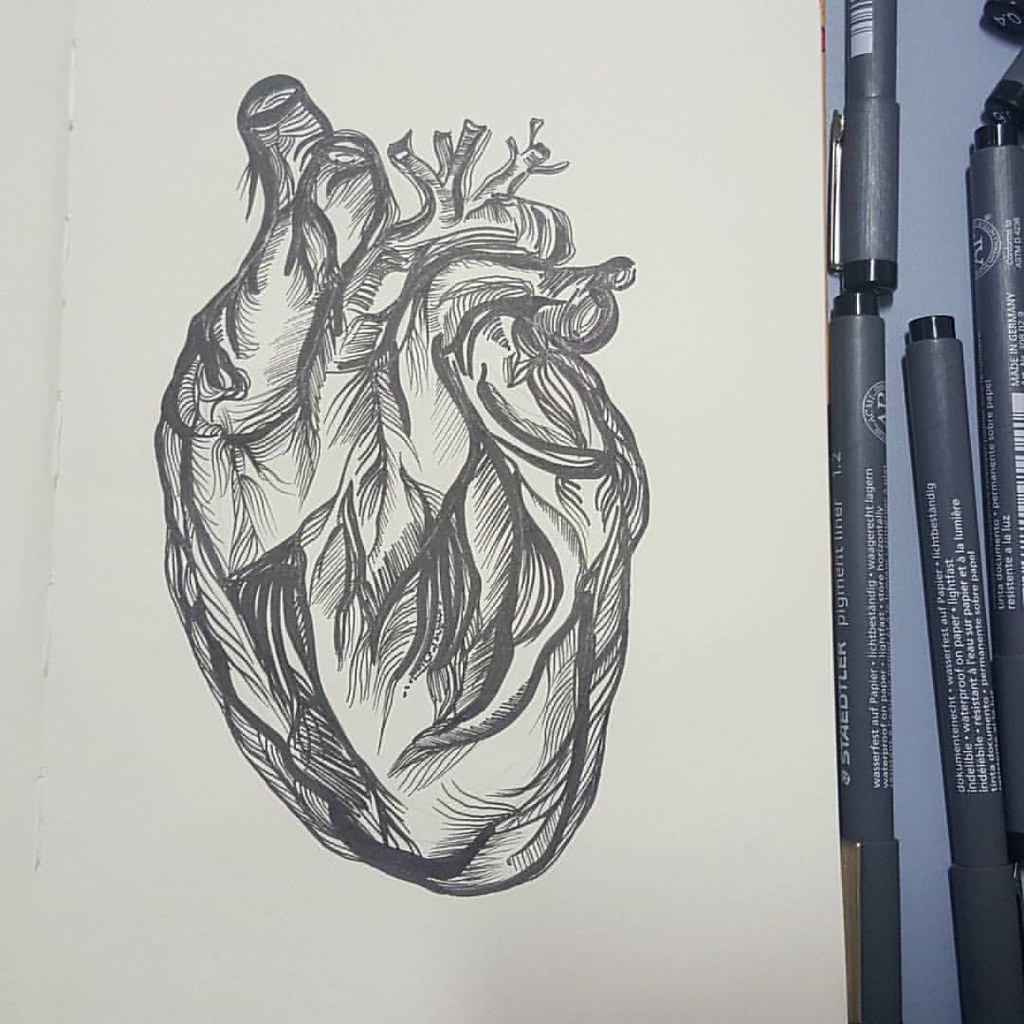An extremely close-up view captures a highly detailed abstract drawing on a crisp white page. Adjacent to the page lies a grayish-blue surface, neatly arranged with around six gray pens. The drawing itself defies easy identification, featuring a blend of bold, sweeping strokes interwoven with delicate, intricate lines. The overall composition resembles a wavy tapestry or perhaps a cluster of leaves. However, a closer inspection reveals a more complicated structure: a rounded base tapering into trunk-like extensions at the top, evocative of an anatomical human heart. The intricate design and rich textures make the artwork visually captivating and thought-provoking.